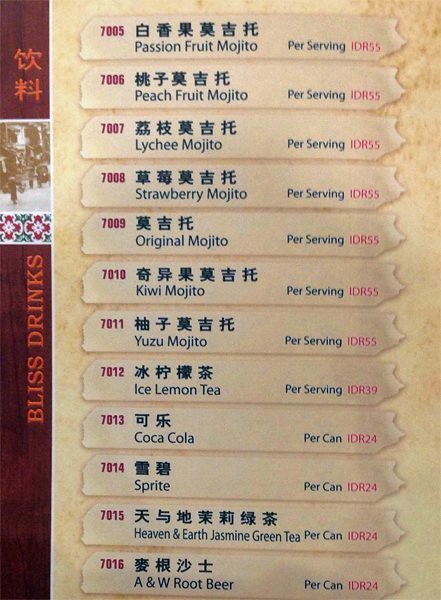The image depicts a rectangular drink menu from an Asian restaurant, with a predominantly cream-colored background. On the left side, a vertical strip, roughly an eighth of the menu's width, features a deep reddish-brown woodgrain texture. At the top of this strip, there are two Asian characters, followed by a blurry black-and-white photo that is difficult to discern. Below the photo, there are green and red floral designs, and vertically written in English, it reads "Bliss Drinks" in all capital letters with red font.

Moving to the right of this strip, the drink options are listed in a beige or tan-colored section. Each menu item is accompanied by a red number, an Asian inscription, and a description in English. The items listed include:

1. **7005 - Passion Fruit Mojito per serving (IDR55)**
2. **7006 - Peach Fruit Mojito**
3. **7007 - Lychee Mojito**
4. **7008 - Strawberry Mojito**
5. **7009 - Original Mojito**
6. **7010 - Kiwi Mojito**
7. **7011 - Yuzu Mojito**
8. **7012 - Iced Lemon Tea**
9. **7013 - Coca-Cola**
10. **7014 - Sprite**
11. **7015 - Heaven and Earth Jasmine Green Tea**
12. **7016 - A&W Root Beer**

Each drink is listed with corresponding red numbers and is interspersed with Asian characters, providing a culturally rich backdrop to the menu.